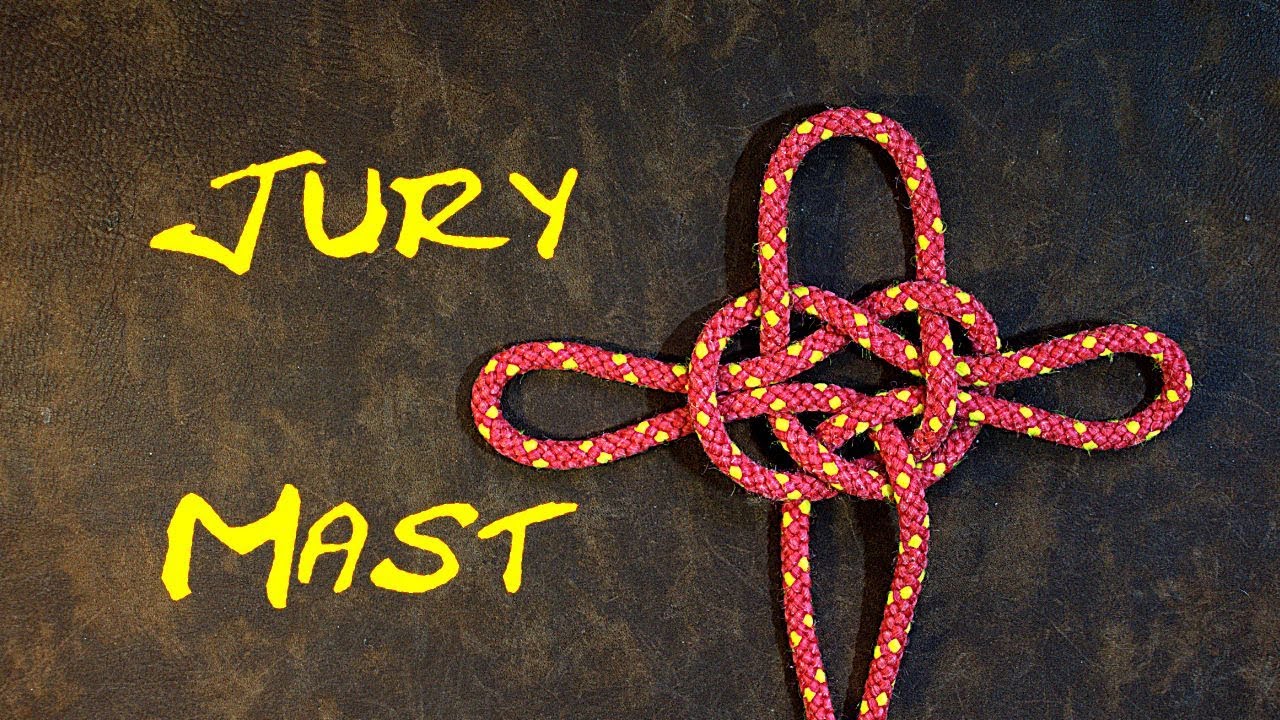The image features an intricately tied nautical knot known as the "Jury Mast," prominently labeled in bright yellow capital letters on the left side of the photo. The background is a worn, appealing, dark brown leather with various shading, giving it a textured appearance. The knot itself is a sturdy-looking maroon rope with yellow spots, arranged in a complex formation. The central part of the knot resembles a pretzel shape with a loop threaded through its middle, creating two additional loops that extend outwards, almost like wings. Below the pretzel section, two rope ends hang down, resembling small legs. The entire knot is laid out flat, showcasing its sophisticated and detailed craftsmanship.